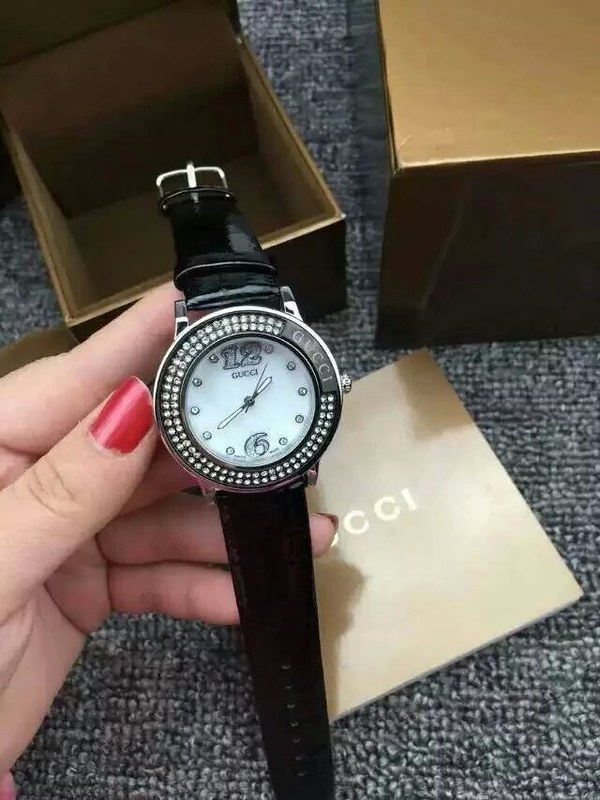The photograph, oriented vertically, captures an elegant hand positioned on the left side of the frame. The person's thumb, adorned with striking red fingernail polish, is extended outward as the hand faces the camera in an open gesture. Draped delicately over the wrist is a sophisticated Gucci wristwatch. This exquisite timepiece features sleek black straps and a prominent circular face. The watch face is encircled by two rows of sparkling rhinestones along the rim, adding a touch of opulence. The Gucci logo is prominently displayed on the frame, lending the watch an air of luxury. The watch face itself is minimalist, marked by rhinestones at each hour, except for the numerals 12 and 6, which stand out for clearer readability. The time shown on the watch is approximately 2:40.